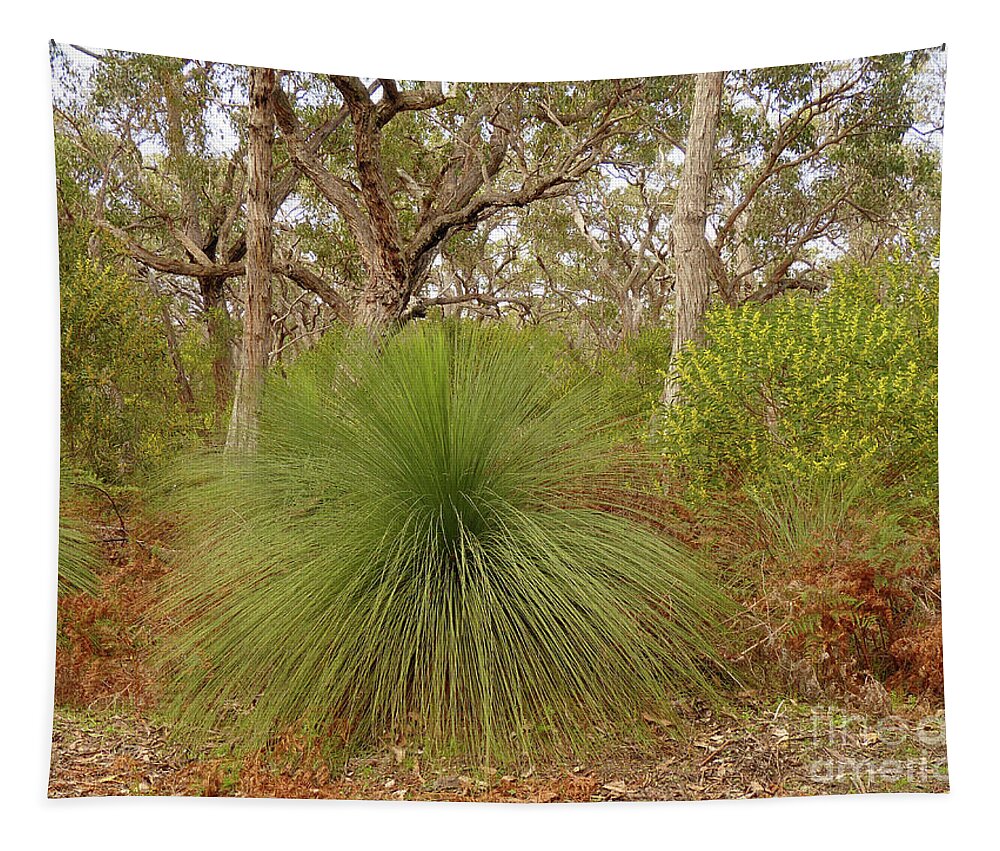This is an outdoor daytime image featuring a variety of bushes and plants arranged in a roughly rectangular-shaped outline, with the top edge dipping from the top left to the right and the middle rising slightly back to the right. The sides are irregular, and the bottom edge appears mostly straight with a slight curvature in the middle. At the bottom of the image, the ground is dirt-covered with leaves and twigs scattered about. 

Dominating the middle-left portion of the image is a distinctive, green, starburst-like plant with thin, wispy leaves that radiate in all directions, giving it a spiky and poofy appearance. To the right of this central plant, there is a small bush featuring slender stems topped with light yellow flowers. 

Further to the left, partially off-frame, another plant similar to the central one is visible. Surrounding these primary plants, the background is filled with a variety of trees. Near the center-left stands a large tree with many branches, flanked by a couple of smaller trees on either side. In the distant background, additional trees frame patches of visible blue sky between their branches.

In the bottom right-hand corner of the image, faint, barely distinguishable white lettering can be seen, with "America" possibly discernible at the bottom. Overall, the scene gives a woodsy feel, suggesting it could have been taken in the fall.